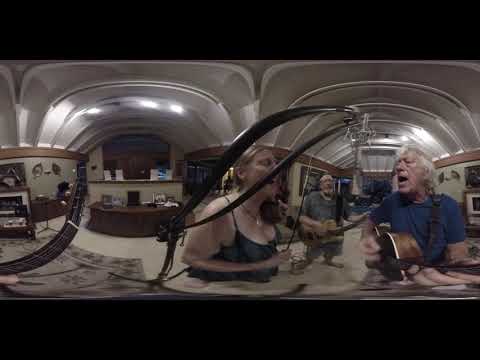The image is a somewhat distorted indoor scene framed by thick black borders at the top and bottom, depicting what appears to be three musicians passionately engaged in a musical performance. On the right side of the image, a man with white hair and a blue shirt is playing a right-handed guitar, with his guitar strap over his neck and his left hand notably distorted. His mouth is open, suggesting he is also singing. Slightly to the left of him, another man in a greenish shirt, possibly barefoot, also seems to be playing a guitar or ukulele, though the instrument is harder to discern due to distortion. In the center left, a woman with blondish hair wearing a black top is playing a fiddle or violin, the bow held in her right hand, and she too is part of the vocal harmony as her mouth is open. 

Behind the musicians, elements of the room, which might be a recording studio or living room, are visible, including pale green walls with posters and pictures, a curved ceiling, and various pieces of electronic equipment and music stands. The scene has an otherworldly and somewhat chaotic visual quality due to the distortion, with some areas appearing more blurred, especially the figure in the background. The left third of the picture reveals a desk cluttered with paraphernalia but no additional figures. This evocative image captures the energetic and passionate atmosphere of the musicians deeply immersed in their performance, despite the surreal distortion of their surroundings.